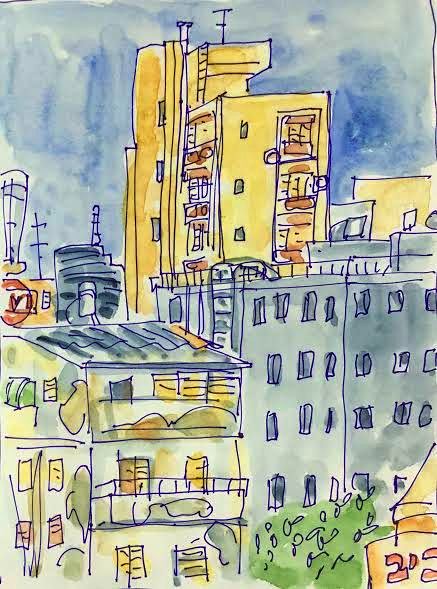This image is a detailed watercolor and pen-and-ink painting of a cityscape, captured in a vertical format. Dominating the scene, a tall, bright yellow high-rise building with many balconies stands prominently in the middle. To its right, there is a grey building with several windows, and below it, a patch of green grass is visible. On the far left, a lighter brown building can be seen next to a greenish-grey structure with windows, railing, and a grey roof. Behind this building, a dark grey canister and a TV antenna can be spotted perched atop another brown building with a peaked roof. Adding to the vibrant details, a lower blue building featuring a ladder and a multicolored building with a tile roof are also depicted. The sky above exhibits a blue-white gradient, and green bushes adorn the bottom of this meticulously crafted urban scene.